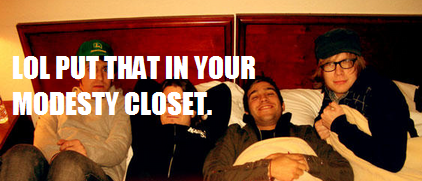This photograph, possibly a magazine clipping, features the band Fall Out Boy. It captures the four bandmates lying side-by-side in a hotel bedroom setting. The beds, seemingly two twin beds pushed together, have cherry wood headboards against a tan or yellowish wall. A matching cherry wood bedside table with a cup on it is visible next to the bed. The men, dressed in jackets and sweatshirts, look to be in their late 20s or 30s. The man on the far left wears a green hat and a gray sweatshirt, while the second from the left is in a black hoodie with hands over his head. The third man sports a green coat over a black hoodie, and the fourth, wearing a black hat and black-framed glasses, has white on his hoodie. White pillows and some sheets partially cover them. Most are smirking or smiling at the camera, especially the man second from the right. Superimposed on the image is the text "LOL PUT THAT IN YOUR MODESTY CLOSET" in all-caps white sans-serif font.